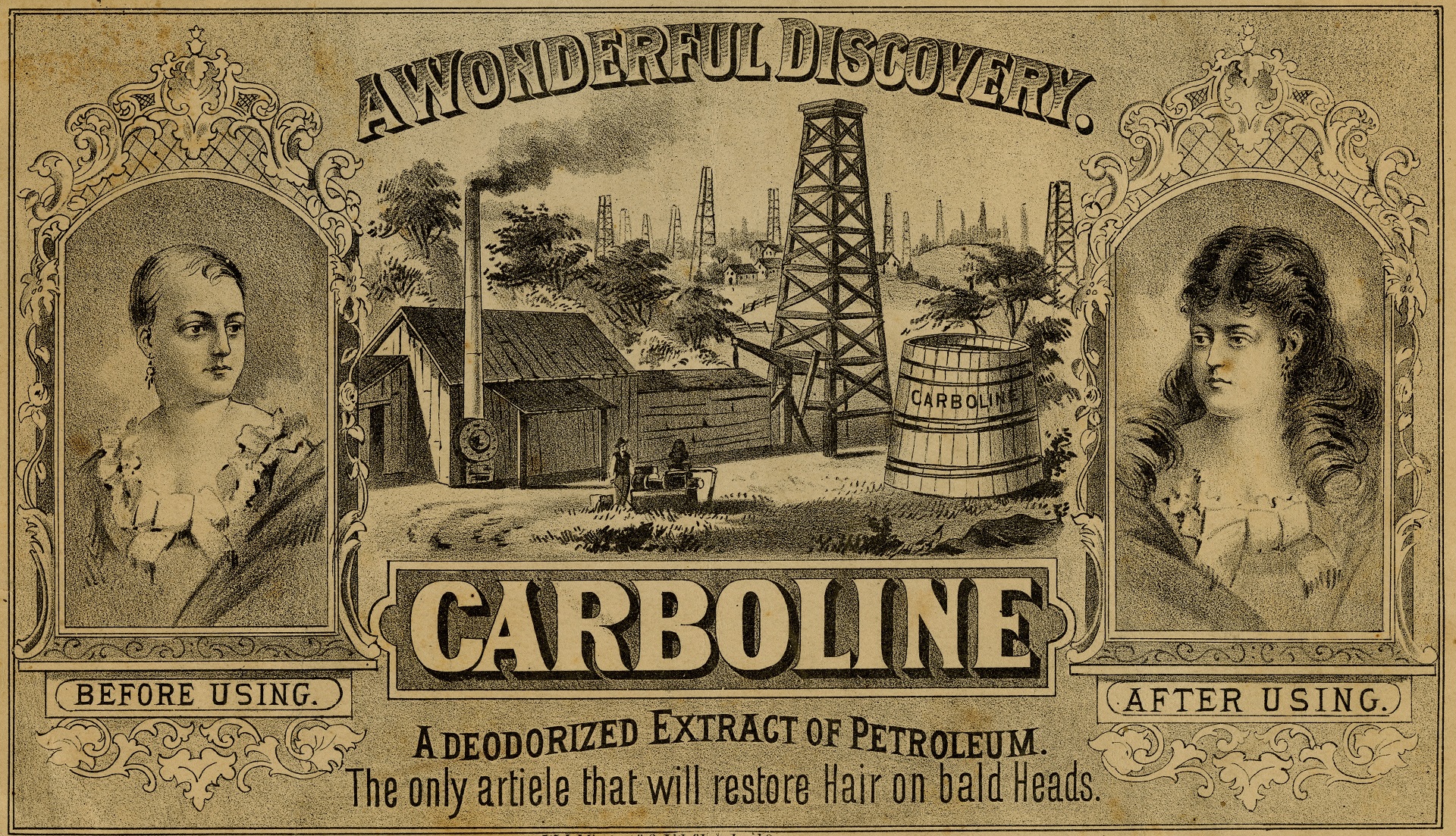The horizontally aligned rectangular image is an old-time advertisement with a light to medium brown, slightly yellowed background. Dominated by black and white illustrations, it features two framed photographs of women, each styled as though seen through a decorative window with an arched top.

In the photograph on the left, there is a woman with short hair wearing an old-style gown with ruffles on the front; the caption underneath reads "before using." The photograph on the right depicts the same woman now with long brown hair and a bow tied to the front of her gown, captioned "after using." 

Across the center of the ad, in prominent block letters, it declares "A Wonderful Discovery." Below this, an illustration showcases a small barn, a windmill, and a barrel labeled "Carboline." Another block-letter text, centered at the bottom, reads "Carboline." The smaller text below asserts, "A deodorized extract of petroleum. The only RTL that will restore hair on bald heads." This piece of artwork, combining both text and imagery, effectively conveys the promise of hair restoration.